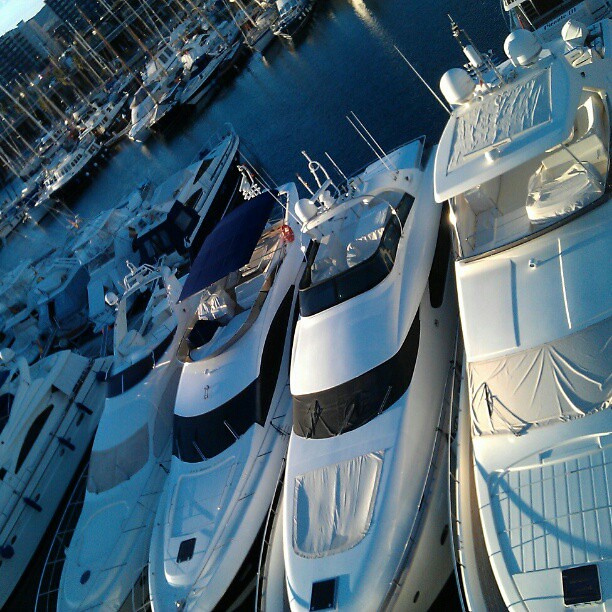This color photograph captures a marina teeming with expensive boats, shot from a peculiar diagonal angle that looks down on the scene. The foreground features four prominent, high-end motorboats, primarily white with some black and blue accents, boasting antennas and electronic equipment housings. These boats are tightly packed side by side in the slips, exemplifying millions of dollars worth of floating luxury. In the mid-ground and upper left corner, rows of additional boats—sailboats discernable by their masts—extend towards buildings that line the marina. The water, visible in patches between the boats and along the left side of the image, appears dark, suggesting either evening light or deep blue hues. The backdrop includes more densely packed boats and possibly a large structure of dark stone with some lighter elements, partially visible beneath an almost entirely cropped-out blue sky. The overall impression is one of immense wealth and sophisticated maritime technology densely packed within a bustling marina.